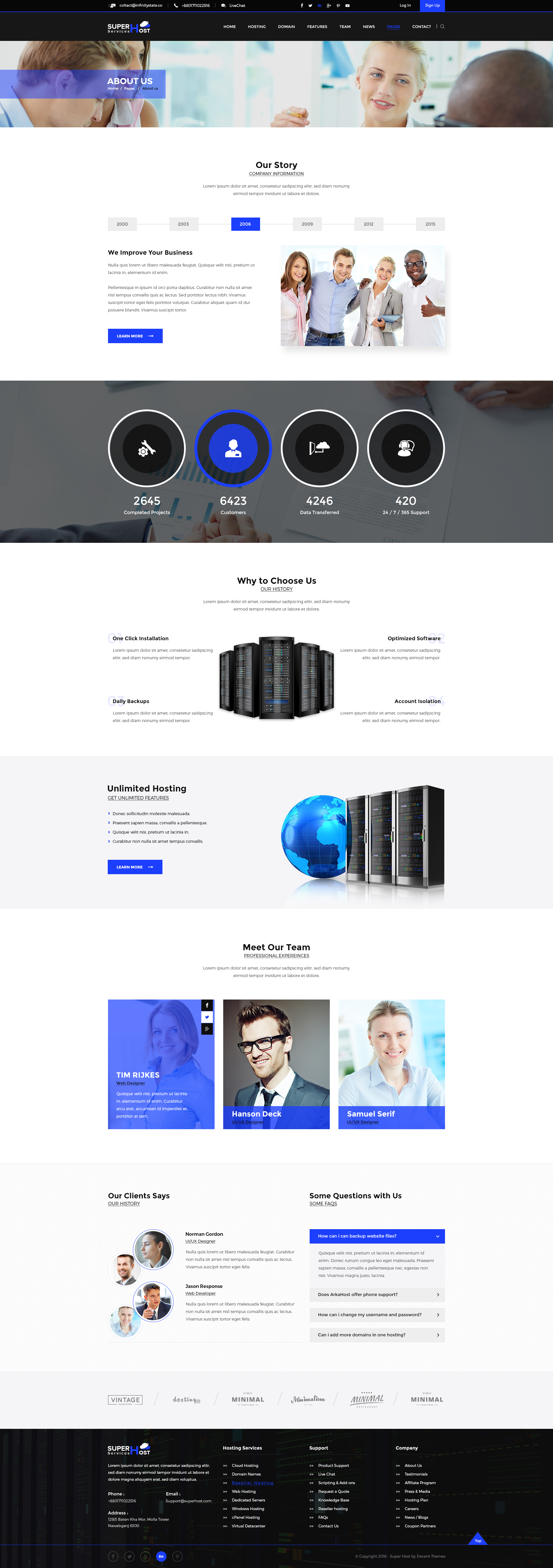The image features a web page with intricate details positioned strategically throughout. At the top, there is a small text banner that reads "Super Host," followed by menu items labeled "About Us," "Our Story," and "Company Information." 

Beneath this, there is a timeline presented in boxes highlighting key years: 2000, 2003, 2004, 2009, 2012, and 2015, accompanied by the slogan "We Improve Your Business." Below the timeline, a photograph captures four individuals posing and smiling at the camera, radiating a professional yet friendly demeanor.

Further down, are several circular icons accompanied by specific statistics: 
- A circle with a wrench and gear icon indicating "2645 Completed Projects."
- A blue circle with a person icon denoting "6423 Customers."
- An icon depicting a cloud with an arrow detailing "4246 Data Transferred."
- Another person icon, this time with a headset, conveying "420 - 24/7/365 Support."

The bottom portion of the image includes a section titled "Why Choose Us?" and lists significant features:
- Our History
- One-Click Installation
- Daily Backups
- Optimized Software
- Account Isolation
- Unlimited Hosting
- Get Unlimited Access

Each of these components is meticulously organized to provide a thorough overview of the company's capabilities, achievements, and services offered.